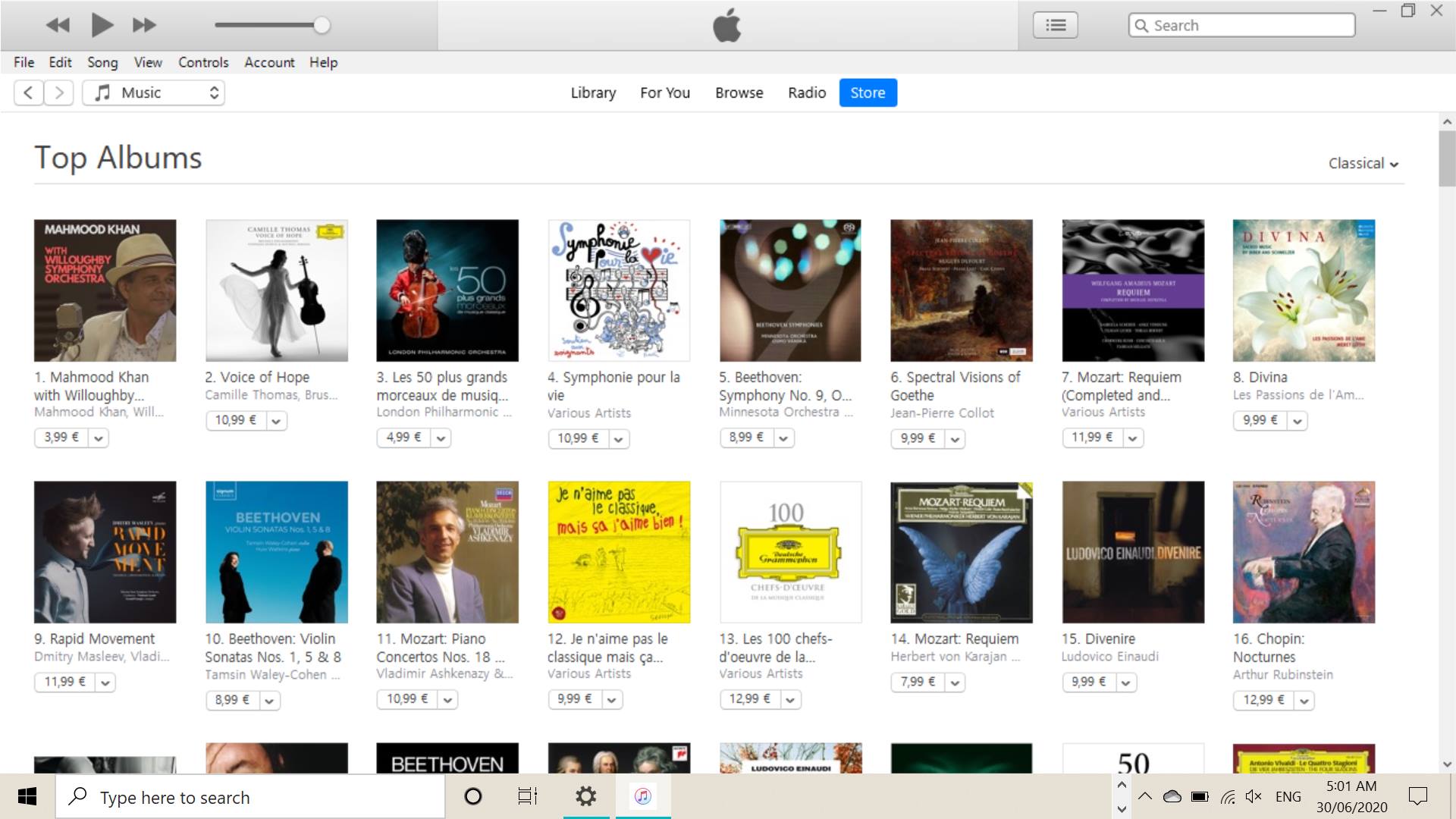The screenshot depicts an Apple webpage, likely Apple Music, due to the prominent Apple logo centered in the top navigation bar. On the left side of this bar, there are standard media controls including rewind, play, and fast-forward buttons, accompanied by a slider bar. The logo "Apple" is prominently displayed in the center.

To the right, there is an information button, a search bar with the placeholder text "search," and standard window control buttons for minimize, maximize, and close.

Directly below the navigation bar, a horizontal menu lists options "File," "Edit," "Song," "View," "Controls," "Account," and "Help." Further below, another navigation section shows directional buttons (left and right), and a label "Music" with up and down arrows on the right side.

In the middle section, there are tabs labeled "Library," "For You," "Browse," "Radio," and "Store." The "Store" tab is highlighted in blue with white text, whereas the other tabs are gray with a white background.

Under this, the main content area displays a section titled "Top Albums" on the left. The section showcases a grid of album covers, consisting of several rows. The visible rows contain the following albums from left to right:
1. "MAHMOODKHAN"
2. "A Voice of Hope"
3. "Less 50 Plus Brands"
4. "Morceaux d'âmsic"
5. "Symphony Pour La Vie"
6. "Beethoven, Symphony No. 9"

A vertical scroll bar on the right side indicates that there are more albums available for browsing. The cursor is positioned on this scroll bar, implying the option to navigate further down the page.